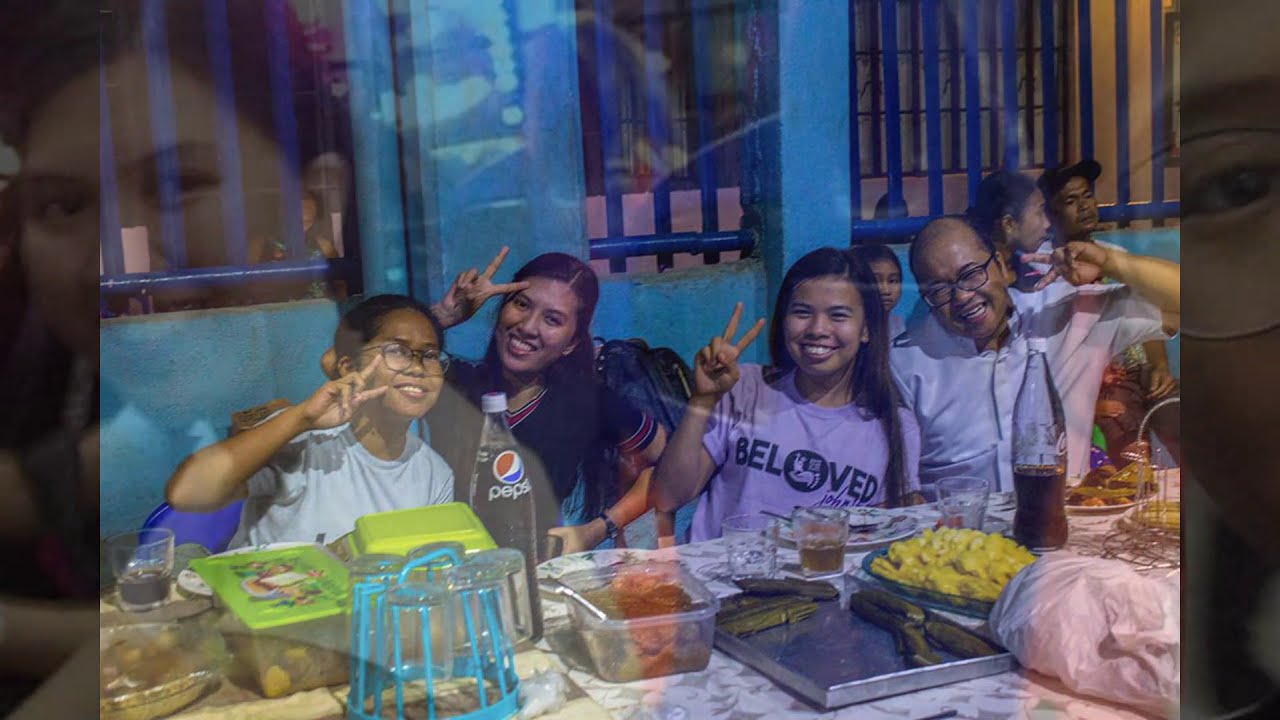In the foreground of the image, four individuals, all holding up peace signs, are seated behind a table laden with a variety of foods and drinks. The group appears to be of Asian descent. On the left, a young girl with black hair and glasses, dressed in a blue shirt, is joined by another young girl with dark hair and glasses, also in a blue shirt. In the center is a young girl with long black hair wearing a gray shirt that says "Beloved." To her right is a nearly bald man donning black glasses and a white button-up shirt. In front of them, the table is filled with an assortment of food, including a silver tray with green pickles, a blue tray with yellow noodles, and a bottle of Pepsi along with other beverages and dishes.

The background features a light blue wall with windows fitted with dark blue bars. There is a reflection in the window, which shows a woman's face with black hair parted down the middle on the left side and an eye with glasses with thin black rims on the right side.

Overall, the scene depicts what appears to be a family enjoying a meal, possibly at a restaurant or a catered event. The atmosphere is lively with the reflection in the background adding a layer of complexity, giving the image a double-exposure effect.